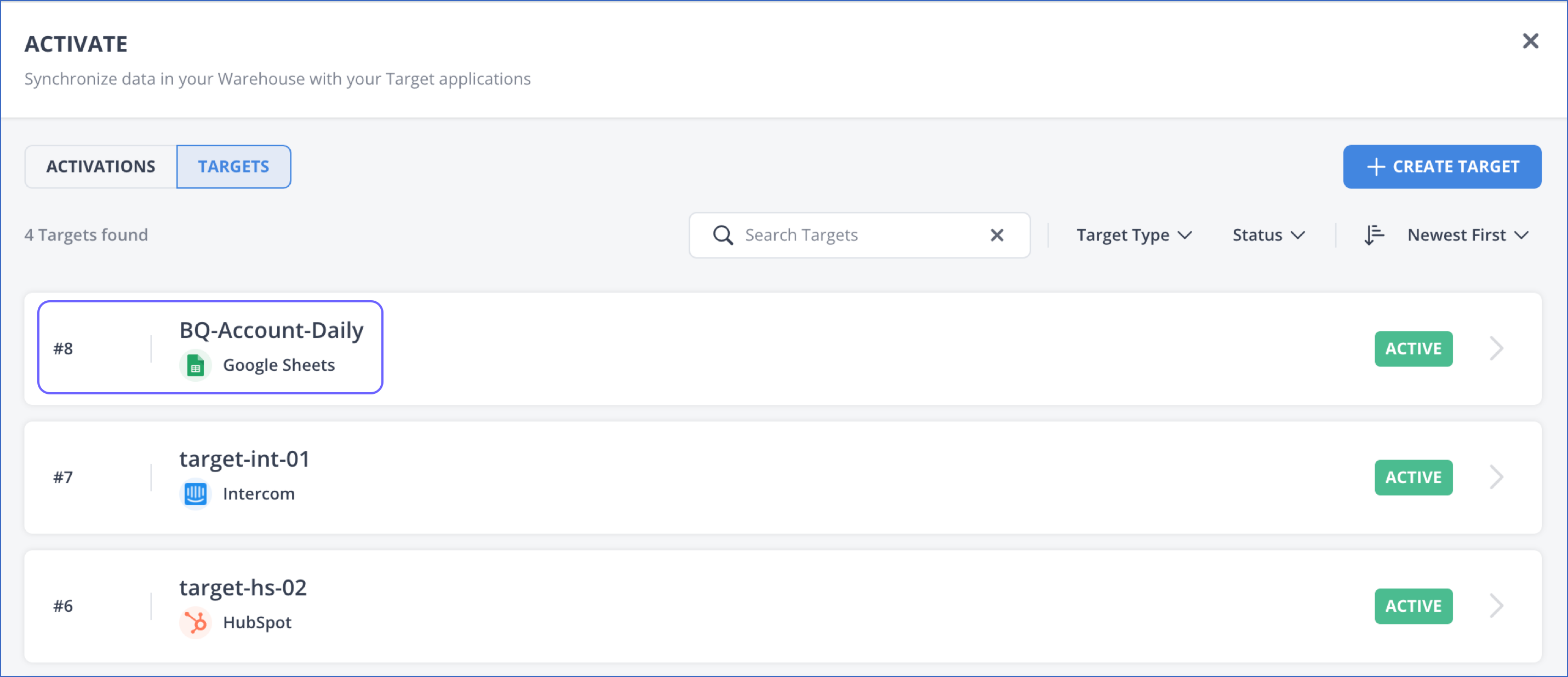This image features a minimalist interface with a white background. In the top-left corner, it says "Activate." Below this, the text reads: "Synchronize data in your warehouse with your target applications."

Beneath this text, there are two tabs. The tab labeled "Activation" is unselected, while the "Targets" tab is highlighted with a blue border, and the word "Targets" is also in blue.

On the far right, there is a blue button with white text that includes a plus symbol and the words "Create Target."

Below this section, it states, "4 targets found." In the center, there is a button labeled "Search Targets." To the right of this are three drop-down menus: "Target Type," "Status," and "Newest First."

Three targets are listed below these menus:
1. The first target is labeled "No. 8, BQ Account Daily Google Sheets," with its status shown as "Active" on the far right.
2. The second target reads "No. 7, Target INT-01 Intercom" and is also marked as "Active."
3. The third target says "No. 6, Target HS02 HubSpot," with its status noted as "Active" as well.